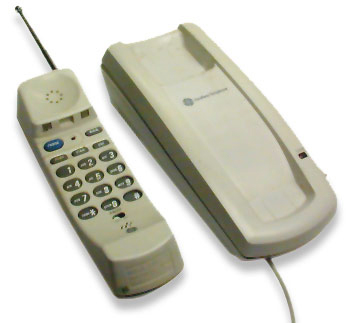This is a detailed photograph of a vintage cordless home phone, likely from the 1990s or early 2000s. The phone is predominantly white and consists of a handset and a base unit, both marked with the GE logo. The handset, lying flat to the left of the image, features a silver extendable antenna that protrudes from the top, and a distinctive blue talk button. The phone's keypad includes the numbers 0-9, as well as the star (*) and pound (#) symbols. The base unit, also white, includes a charge indicator light on the right-hand side and has both a power cord and a phone connection cord visible at the bottom. The phone is positioned in such a way that the antenna, earpiece, mouthpiece, and numeric keypad of the handset are clearly visible. It appears to be set on an indeterminate surface against an all-white background, giving the impression that it is floating without any discernible environmental context.